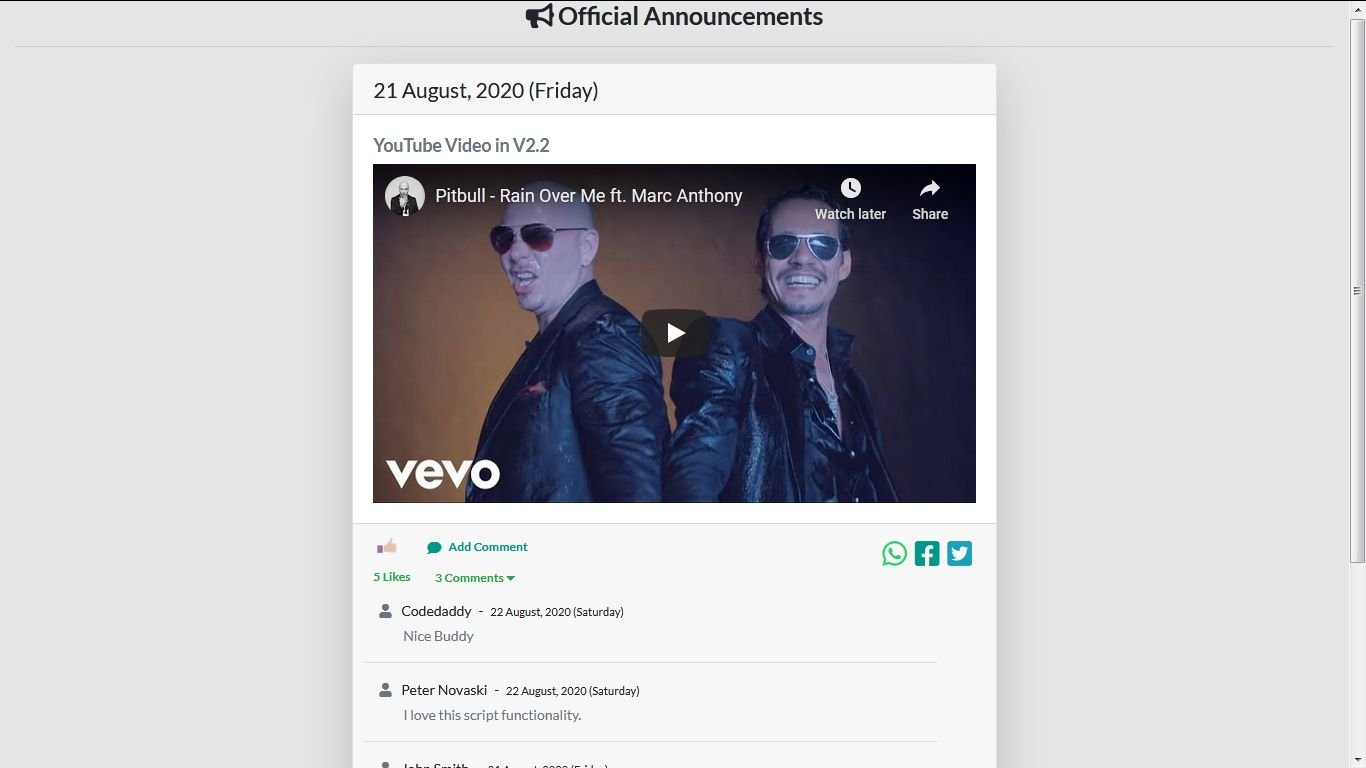The image appears to be a screenshot from a digital device, possibly a computer or smartphone. The background is gray, and prominently featured in the center is a white rectangular box. At the top of the gray background, the text "Official Announcements" is displayed in black, accompanied by a megaphone icon to the left.

Inside the white rectangular box, the date "21 August 2020 (Friday)" is listed at the top. Below that, the text reads "YouTube video in V2.2." Dominating the center of the rectangle is a video thumbnail, which includes text at the top stating "Pitbull - Reign Over Me (featuring Marc Anthony)." To the left of this text is a circular icon with an image of a bald man.

The thumbnail shows two men wearing sunglasses and leather jackets. The man on the left is bald and facing to the left with his mouth open, while the man on the right has black hair, a darker complexion, and a mustache, facing forward with a smile. There is a play button centered between the two men. At the bottom left of the thumbnail, the VEVO logo is visible. 

The screenshot also includes the beginning of a comments section at the bottom. The first comment is from a user named "Code Daddy," who says, "Nice buddy." The second comment is from "Peter Nowinski," who states, "I love this script functionality." 

In the upper right corner of the thumbnail, options to "Watch Later" or "Share" are displayed. This detailed view captures the essence of an interactive media post featuring a music video announcement and community interactions.